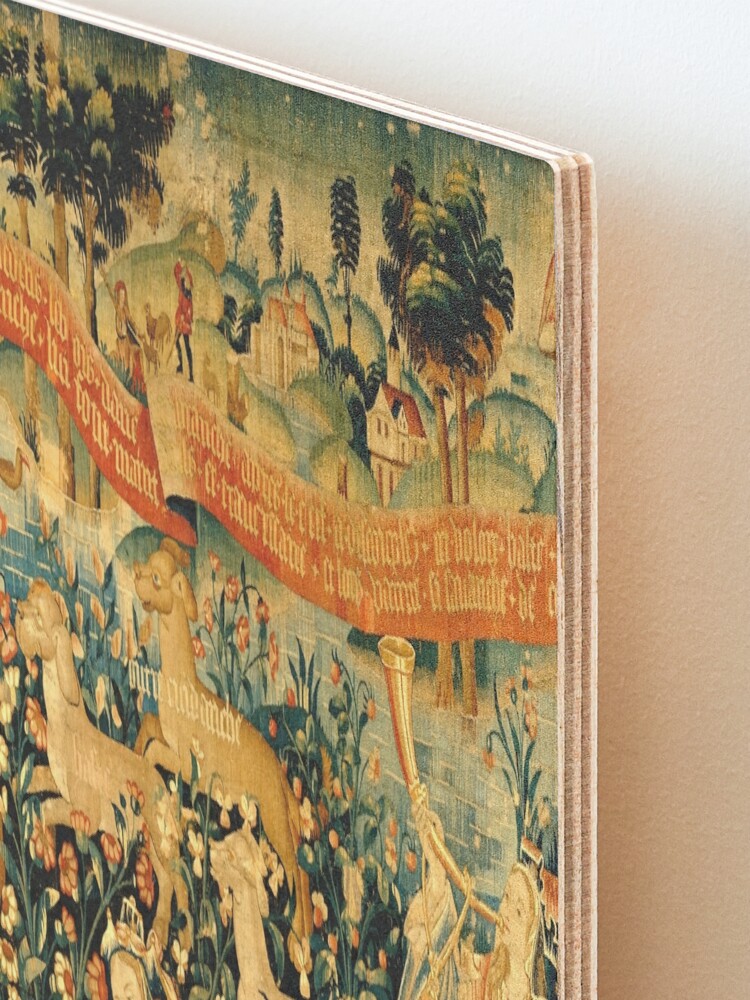The image depicts a busy medieval scene printed on a rectangular wooden panel comprising several layers of wood glued together. The painting, occupying about 75% of the image, is angled downward, revealing the board's thickness and creating a triangular section of off-white wall on the right. The artwork features a vibrant and detailed medieval tapestry-like scene. 

In the foreground, a woman in medieval dress blows a long, curved outdoor horn, her figure partly visible from the shoulders up, positioned in the bottom right corner. Two light brown dogs with cartoonish features stand in a field of vivid red and pink flowers. A prominent orange banner with ornate, hard-to-read white text, possibly in Latin, stretches across the middle of the scene, with a small body of water and a resting duck beneath it.

The background showcases a picturesque landscape with tall, hilly terrain dotted with about seven trees and several houses. Among the flora, there are churches and other buildings, creating a quaint medieval village atmosphere. Scattered throughout the scene are various individuals, including a shepherd with sheep near the upper left. The sky transitions from light near the horizon to a darker blue overhead, adding depth to the pastoral vista.